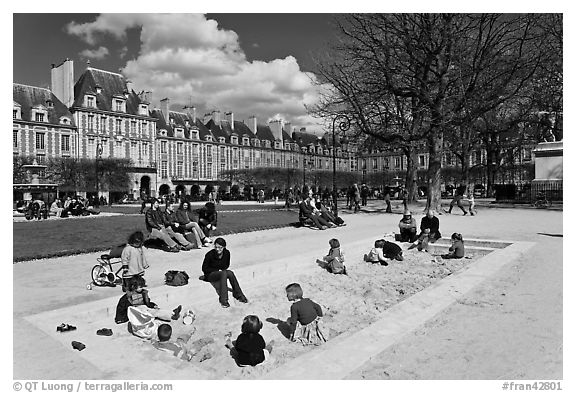This black-and-white photograph captures a serene scene of children playing in a large concrete sandbox, supervised by a few adults seated at the edges. The children, dressed in long sleeves, appear to be fully engaged in their play, and there is even a child with a bicycle nearby. Surrounding the sandbox, several adults are seated on park benches, all donned in long sleeves and long pants, hinting at a cool day. Behind the benches, a strip of grass borders a vast, old European-style building that stretches across the background, turning at a 90-degree angle. This historic-looking structure, adorned with pillars, suggests a school, business, or university. On the right side of the image, a tall, bare tree without leaves stands prominently. Above the scene, a cloudy sky completes the picturesque moment. At the bottom of the photo, a watermark reads "copyright QT Luong/Tara Galleria.com," alongside the hashtag "Fran 42801."